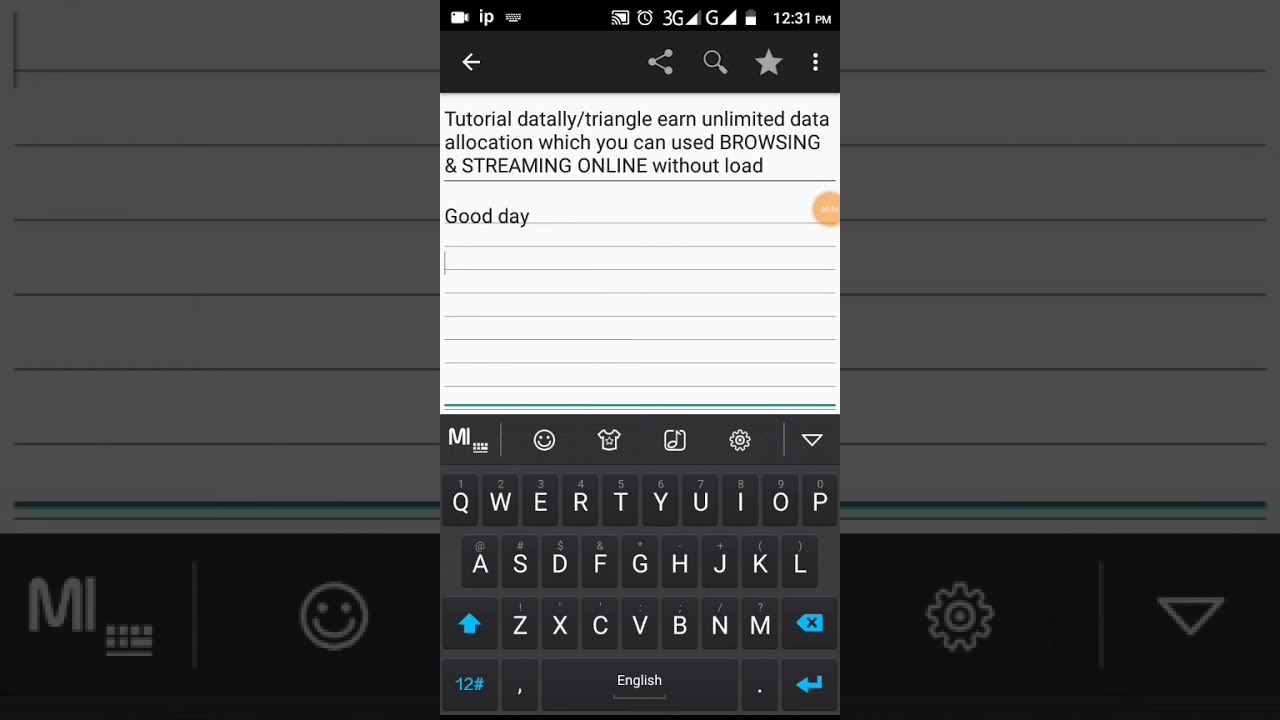This is a highly detailed horizontal image depicting a digital environment one might encounter when using a messaging application on a computer or tablet while multitasking. The background of the image resembles grayed-out lined paper, lending a subtle, organized appearance. In the lower left corner of this area, “MI” is displayed beside a keyboard icon, followed by a smiley face.

Overlaying the grayed-out background is a pop-up menu that appears to be part of a messaging app interface. Adjacent to this main image, a settings icon and an upside-down triangle can be seen, likely indicating further customization options.

The messaging app pop-up includes a top bar with a video recording IP displayed alongside various icons. These icons include a left-facing arrow, a triangle with dots, a search magnifying glass, a star, and an ellipsis (three dots), likely serving different functional shortcuts.

Below this top bar are the words: "tutorial, dataly, triangally, triangle, earn unlimited data, allocation which you can use browsing and streaming online without load." 

Further down, the message "good day" appears in an area resembling lined paper, and beneath it lies a QWERTY keyboard, replicating the symbols seen at the bottom of the grayed-out background area. The QWERTY keyboard enhances the interactive feel, suggesting active communication. 

Overall, the image illustrates a snapshot of a digital workspace where messaging and various functionalities blend seamlessly into the user's workflow.